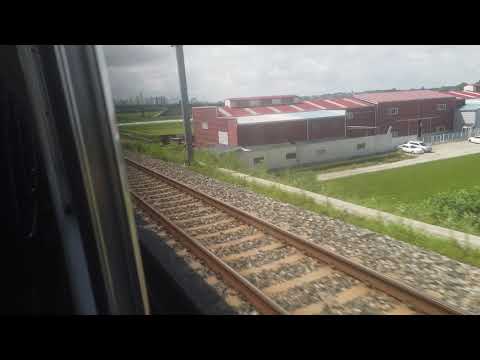This photograph, taken from inside a train, captures a detailed outdoor scene of a train depot area. The image includes a portion of the train window, with a visible metallic border on the left side and a black bar at both the top and bottom edges, framing the view. The foreground features parallel brown train rails running diagonally from the center left to the bottom right of the image, interspersed with gravel pathways and cross ties. The outside area showcases a lush ground filled with vibrant green grass.

In the mid-ground, there's a prominent large red building, possibly resembling a rodeo or fairgrounds structure, stretching from the center left to the right of the image. Near this building, various white vehicles are parked, and fencing is evident around the perimeter. The distant background is characterized by additional buildings set against a hazy, gray, cloudy sky, contributing to the overall atmosphere of a typical, overcast day at a train track. The combination of colors in the photograph includes shades of brown, beige, gray, green, red, black, and white, enhancing the vividness and realism of this outdoor daytime scene.